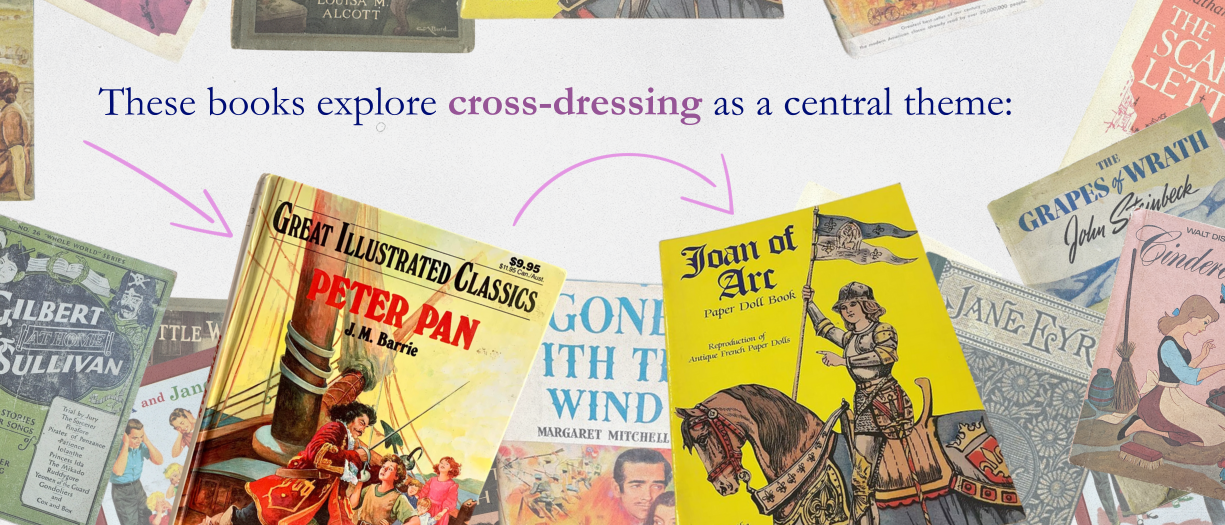The image is a rectangular photograph, approximately six inches wide and two inches high, featuring an overhead view of several book covers laid flat against a surface. Across the top center, there is text on a white background that reads, "These books explore cross-dressing as a central theme," with "cross-dressing" highlighted in pinkish-purple and the rest in blue.

The arrangement of the books starts on the left with titles such as "Gilbert Sullivan," "Little Women," and "Dick and Jane." The most prominent book in the foreground is "Great Illustrated Classics: Peter Pan" by J.M. Barrie, which is accompanied by a pinkish arrow pointing towards it. Behind this, there is a copy of "Gone with the Wind."

Front and center is "Joan of Arc," featuring a yellow cover with a depiction of a lady on a horse holding a flag, also marked by an arrow. To the right of this, partially visible, are "Jane Eyre," "Cinderella," and "The Grapes of Wrath" by John Steinbeck. In the upper right corner, "The Scarlet Letter" can be faintly seen among the collection of book spines. 

The composition and textual emphasis suggest that this might be an advertisement seen in a bookstore or library, highlighting literature where cross-dressing is a significant theme.